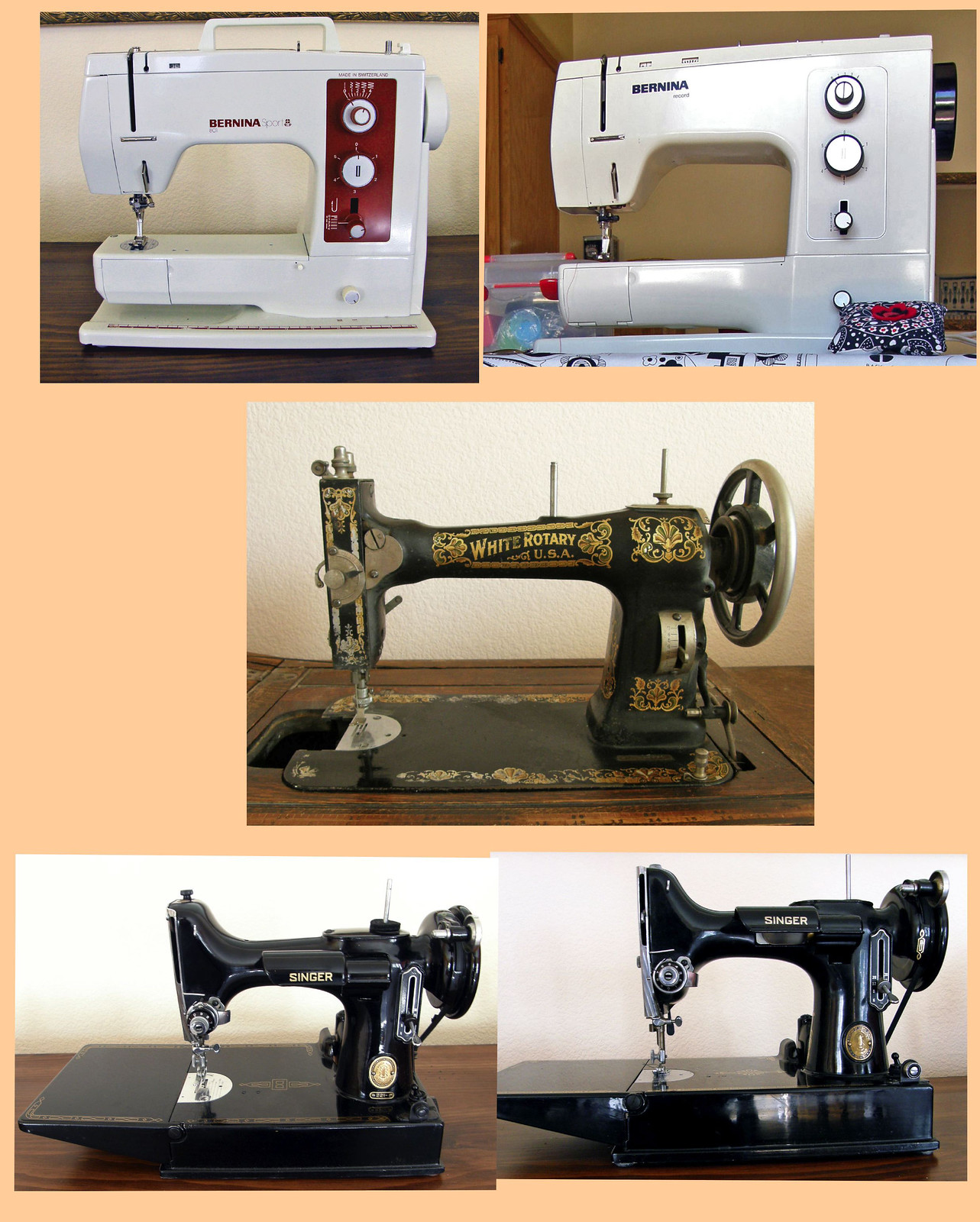This is a detailed color photo collage featuring five different sewing machines set against a plain peach-colored background. The collage is arranged with two images at the top, one in the middle, and two at the bottom, with the photographs varying in size and seemingly placed haphazardly on a computer screen. At the top left, there's a modern, white Bernina sewing machine featuring red trim and a red logo with two stacked buttons on a red rectangle. The top right also showcases a white Bernina sewing machine, this time with blue branding, and additional sewing accessories visible in the frame. Centrally positioned is an antique hand-crank sewing machine by White Rotary USA, notable for its black body with intricate gold decorative patterns and being mounted on an old brown wooden sewing table. Both bottom images display sleek, black Singer sewing machines, adorned with gold and chrome trim, and resting on brown tables. The collage skillfully captures the evolving design and technological advancements of sewing machines through the ages.